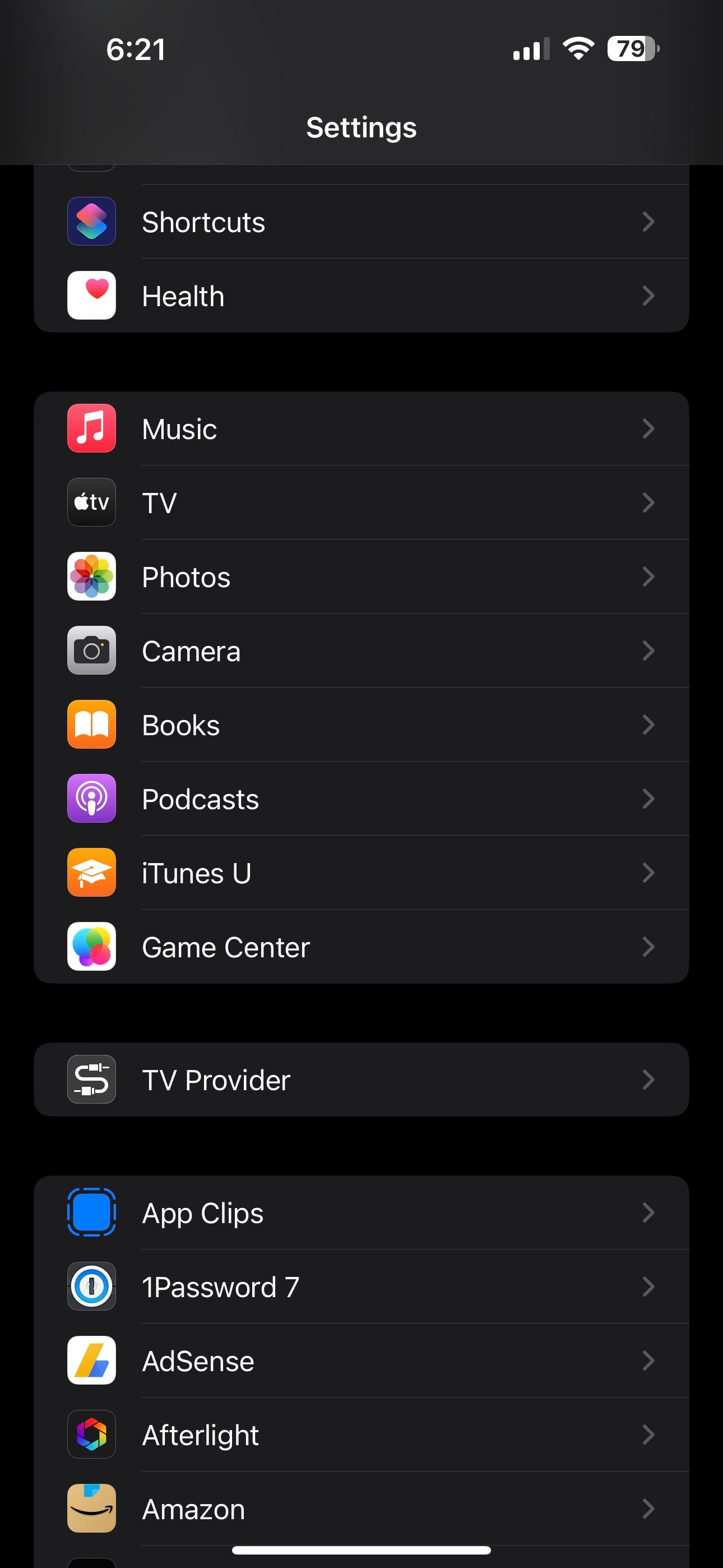Cell phone screenshot with a black background is depicted. At the top, a dark gray rectangle spans across the screen. On the left side of this rectangle, the current time is displayed in white. On the right side, there are icons for reception, Wi-Fi, and battery status. Centered two lines below, the word "Settings" is prominently displayed in white text. 

Below "Settings," there are several boxes with a dark gray background, each divided by light gray lines. Each item listed within these boxes has an icon to its left, a white name label, and a right-pointing gray arrow resembling a sideways 'V' on the far right.

- The first box contains the options "Shortcuts" and "Help."
- The second box includes a variety of media-related options: "Music," "TV," "Photos," "Camera," "Books," "Podcast," "iTunes U," and "Game Center."
- The third box has the single option "TV Provider."
- The final box lists several applications: "App Clip," "1Password" (with the numeral '1'), "7," "AdSense," "Afterlight," and "Amazon."

Each of these items follows the same layout, providing a clean and organized interface for the user to navigate.